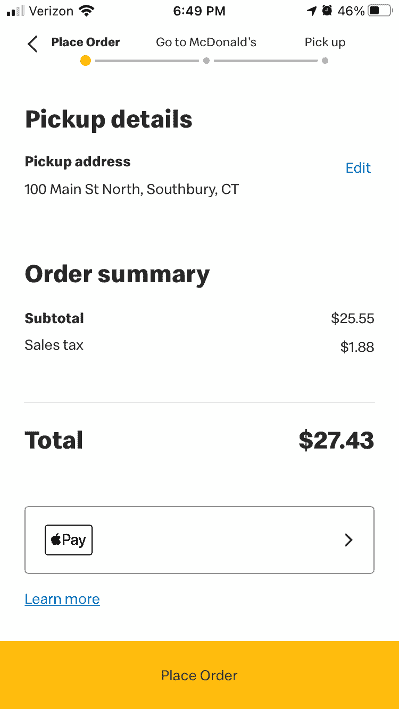The image displays the screen of a Verizon smartphone, indicating it is 6:49 p.m. with a 46% battery life remaining. The focus of the screen is an app showing the pickup details for a food order. At the top section of the screen, a timeline illustrates the progress of the order: a yellow dotted line highlights “Place Order,” followed by a gray line leading to a gray dot labeled “Go to McDonald's,” and another gray line ending at a final gray dot labeled “Pick up.”

The pickup details indicate the address as "100 Main Street North, Southbury, CT," with "CT" appearing in capital letters. Next to the address, the word “edit” appears in blue, suggesting that the pickup location can be modified.

Beneath the pickup information, an order summary is provided. The subtotal of the order is listed as $25.55, with a sales tax of $1.88, making the total $27.43. At the bottom of the screen, options for payment are displayed, including Apple Pay. The prompt “Learn More” is also visible, along with a “Place Order” button highlighted in a yellow rectangle, ready for the user to complete the transaction.